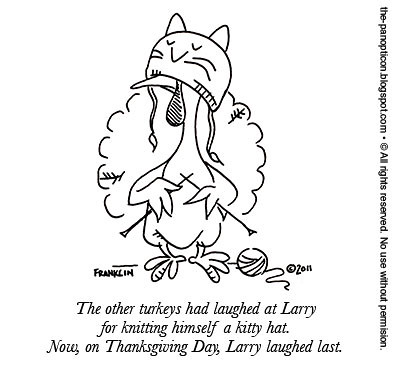This is a black and white sketch of a cartoon turkey named Larry, proudly holding knitting needles while wearing a whimsical kitty hat complete with ears, whiskers, eyes, a mouth, and straps hanging down. There is a ball of yarn on the floor to his right. The caption beneath the turkey humorously reads: "The other turkeys had laughed at Larry for knitting himself a kitty hat. Now, on Thanksgiving Day, Larry laughed last." The artist's name, Franklin, and the date, 2011, are noted at the bottom left of the drawing. Furthermore, running vertically along the right-hand side of the page is a notice reading: "the-panopticon.blogspot.com Copyright all rights reserved. No use without permission."